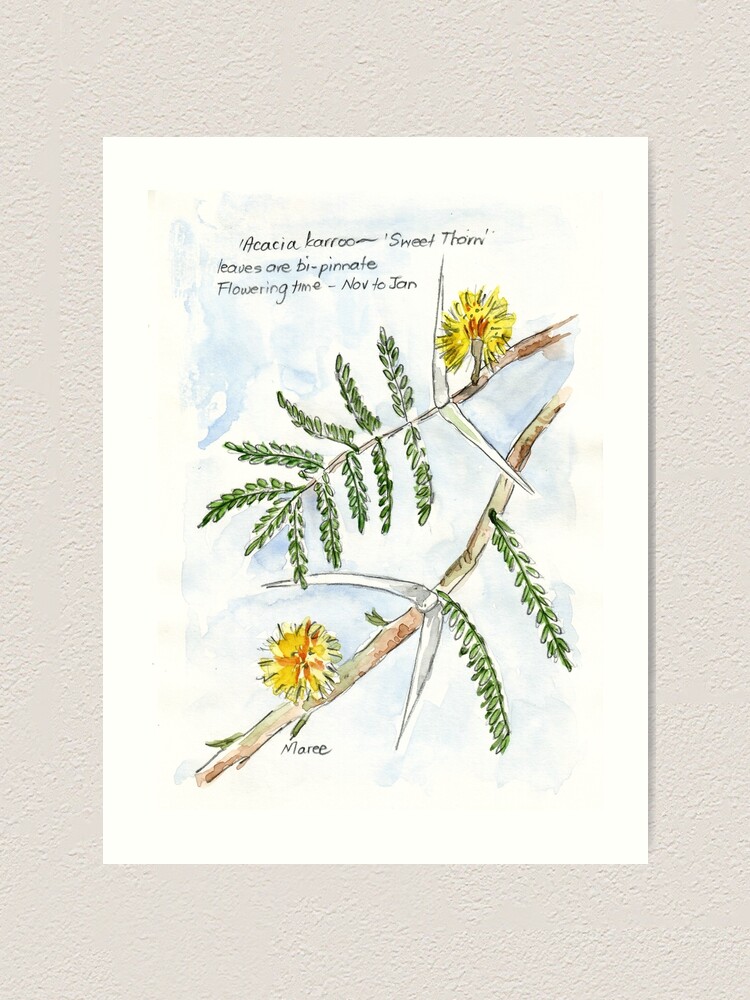This image showcases a delicate watercolor painting of the plant "Acacia Karu Sweetthorn," with its bipinnate leaves and flowering period from November to January. The artwork, labeled "Marie," features two dandelion-like flowers that are yellow with subtle hints of brown and orange, appearing circular and fluffy. These flowers and thin green leaves extend from a larger central stem. The watercolor painting is set against a light blue background, with an unpainted white border. The whole piece is laid against a textured surface of tan color.